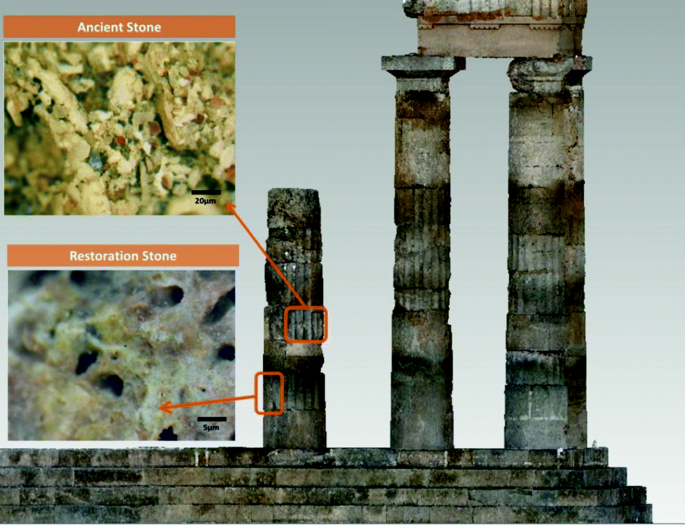In this landscape-oriented image, we see a detailed depiction of ancient classical stone columns, likely from the Greek or Roman eras, set within a ruinous building site. The background reveals two full, weathered columns on the right side, composed of aged stone laden with blacks, grays, and various marks of time. A smaller, partial column stands isolated toward the center, with stone steps visible beneath these structures. An object, possibly a chest or stone frame, connects the two full columns.

On the left side of the image, two color photographs are positioned vertically, each outlined by an orange horizontal rectangle with white text labels. The upper photograph shows a close-up of "Ancient Stone," while the lower photograph details "Restoration Stone." These images highlight the subtle microscopic differences between the original and restored materials. Orange arrows point at specific features on the shorter column, offering a comparative analysis of the stones' textures and compositions. This combination of photographic realism and graphic design effectively illustrates the distinctions between ancient and restored stonework within the archaeological context.